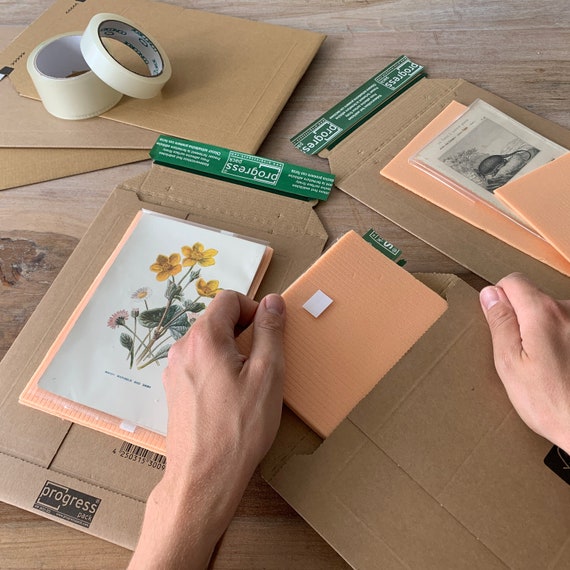In this professionally shot photograph, a pair of white hands, presumably male, is meticulously loading greeting cards adorned with images of flowers, possibly daffodils, into flat, brown cardboard envelopes. The scene suggests someone preparing shipments, perhaps for a small business or an online store. The six visible envelopes appear sturdy, with adhesive strips for secure closure. In the foreground, three envelopes are being actively worked on, each holding a salmon-pink card, while the remaining three envelopes, along with two rolls of tape—one masking and one clear—are stationed in the background on what looks like a wooden surface, possibly a desk or floor. The brand "Progress" is noted on some elements, indicating these items might be part of a "Progress pack".